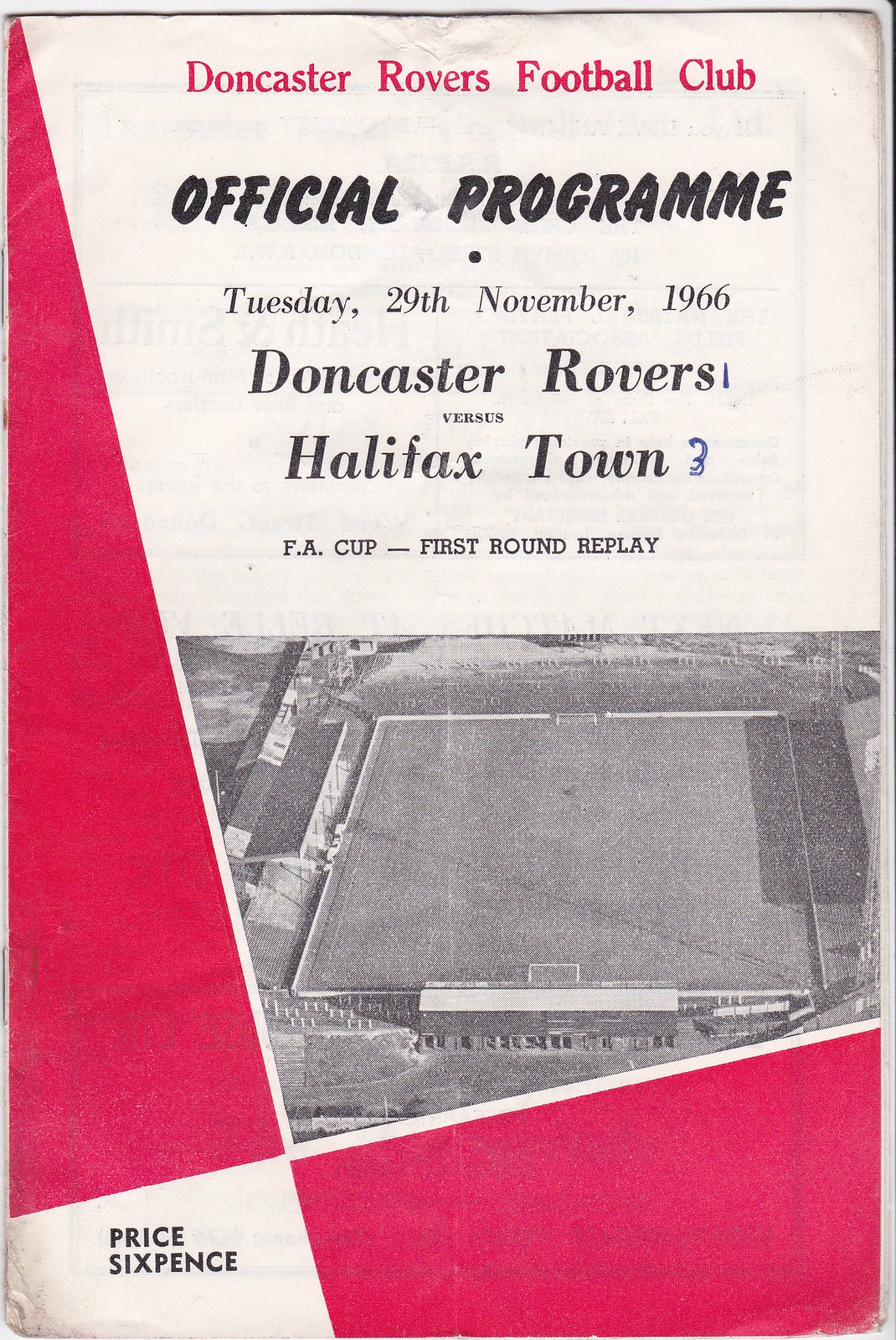This is a detailed, descriptive caption integrating all given inputs:

This is a photograph of an old program from a 1966 football match. Set against a white background, the program features a bold red triangle running vertically along the left edge, accompanied by an asymmetrical four-sided figure in the bottom right corner. The design prominently uses red, white, and black, though the photo is in grayscale with some gray elements. 

At the top, in red letters, is "Doncaster Rovers Football Club" on a white background. Just below, in black letters, it reads "Official Program." The date "Tuesday 29th November 1966" follows, also in black text. Beneath this, it states "Doncaster Rovers versus Halifax Town," and "FA Cup First Round Replay." Handwritten in blue ink next to "Doncaster Rovers" is the number one, and next to "Halifax Town" is the number three, possibly indicating the match score.

A black-and-white photograph of an empty football stadium is displayed under the text. In the bottom left corner of the program, it quietly notes the price: "Price: Six Pence."